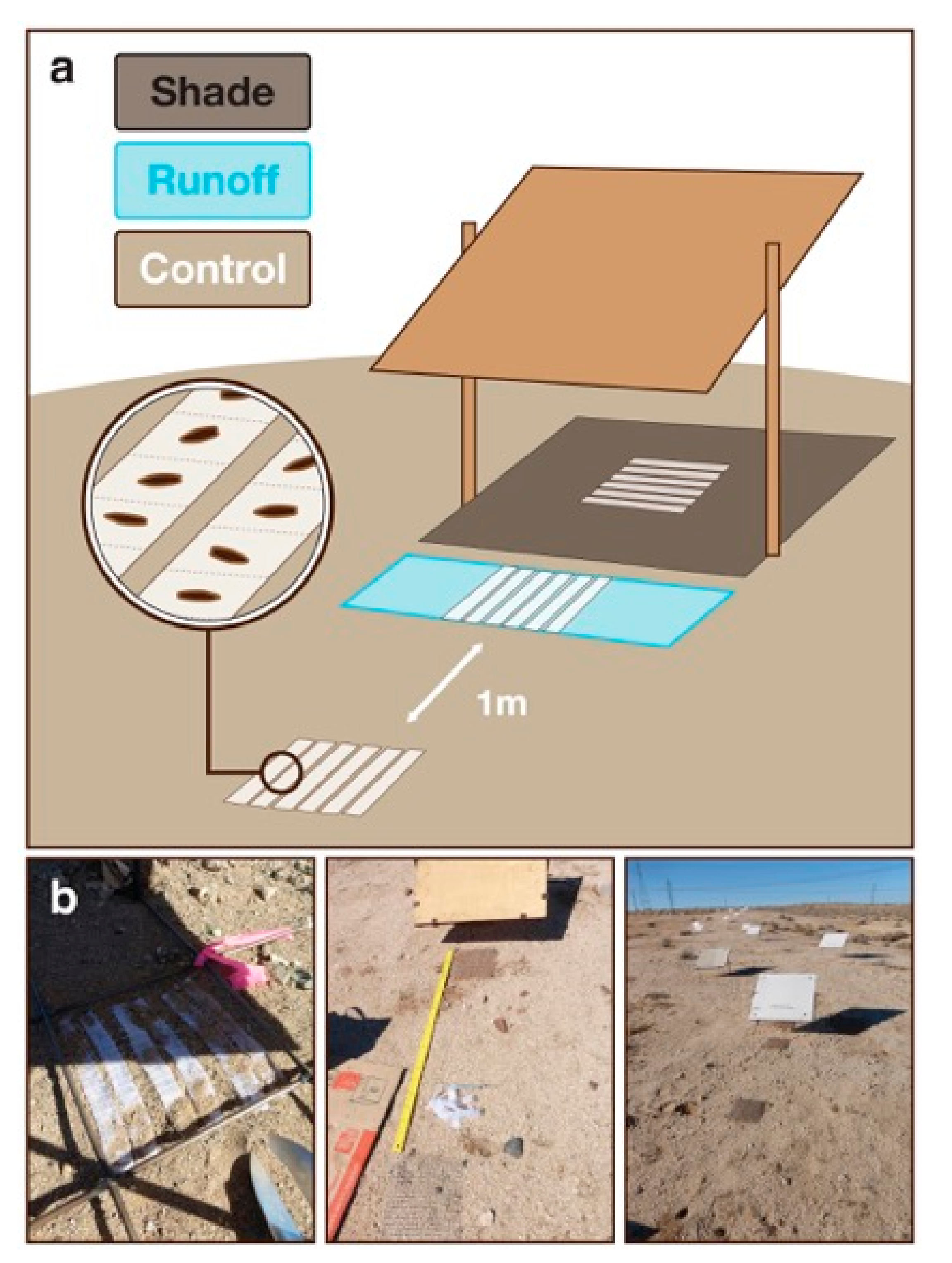The image consists of a detailed illustration and photographs showcasing a method to manage outdoor cultivation involving shade, runoff, and control mechanisms. At the top, a digitally illustrated square outlined in black displays a large, elevated square board providing shade, supported by two brown poles. Various colored rectangles within the square—the brown one labeled "shade," the blue one labeled "runoff," and the beige one labeled "control"—offer a legend to interpret the diagram. Below this diagram, the shaded area contains horizontal white lines, and in front are vertical white lines extending up and to the left.

Adjacent to the right of the diagram, a brown square board hangs diagonally on the poles, above a darker brown square and a blue rectangle with white lines. A magnified circle highlights a detail with brown marks, possibly indicating seeds on white strips embedded in the soil.

Below the diagram, three vertically arranged photographs depict real-life implementation of this method in a desert-like environment with dirt ground and sand. The photos illustrate small square shades erected over various patches of dirt, each with distinct features such as white stripes casting shadows, beige-colored boxes, and white squares laid out on top of the soil.